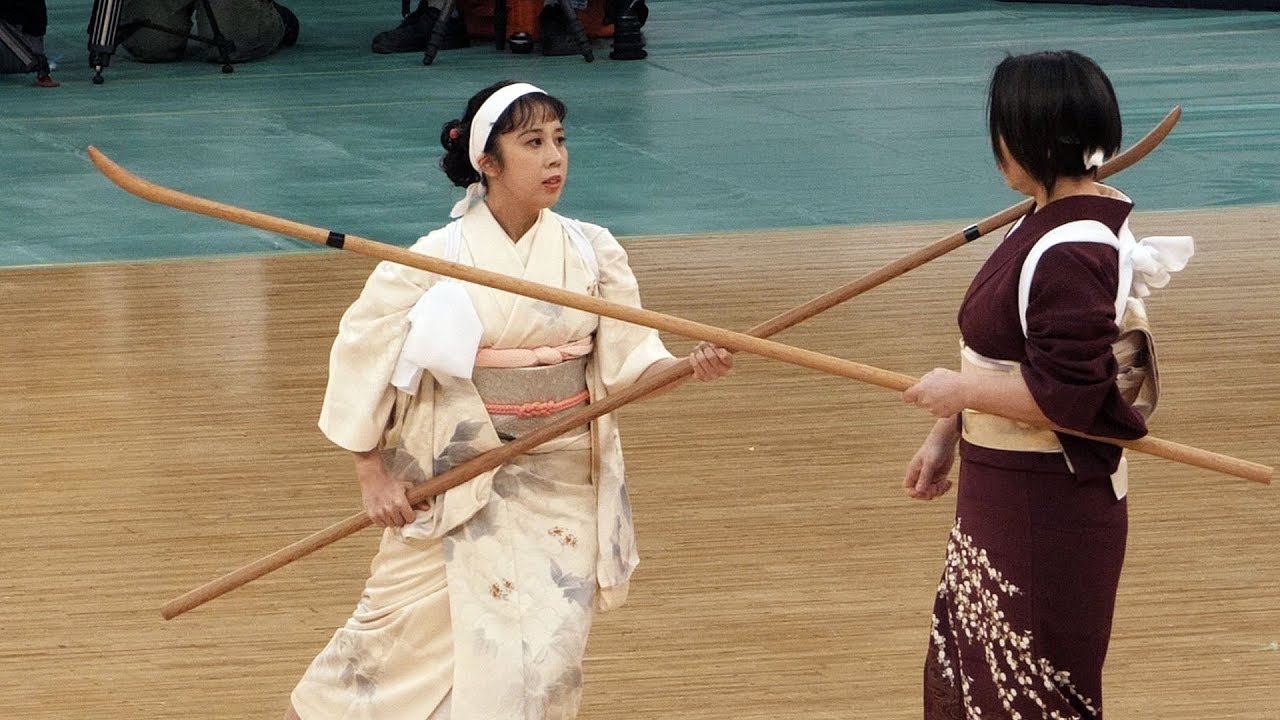The image depicts two Japanese women engaged in a duel-like pose on a glossy beige wooden arena floor, indicative of a tournament setting. In the background, there is a teal blue smoothly-tiled floor. The woman on the left is dressed in an eggshell white kimono with a silvery waistband and a pink knotted obi, complemented by a white bandana over her black, bun-tied hair. She wields a long wooden pole with a curved, pointed end, held with both hands at an angle to the right. The right-hand side of the frame features another woman in a burgundy red kimono adorned with a white floral pattern on the skirt, her medium-length black hair left loose. She holds a similar long pole with her left hand, angled upwards to the left. The curved end of the left woman's pole rests on the right woman's right shoulder, as if they’re poised in a competitive stance, their gazes interlocked. In the background, you can also see various equipment, including tripod legs and red cloths, suggesting a professional setup. Behind the women, blue bean bags are faintly visible, adding to the scene's detailed and cluttered ambiance.